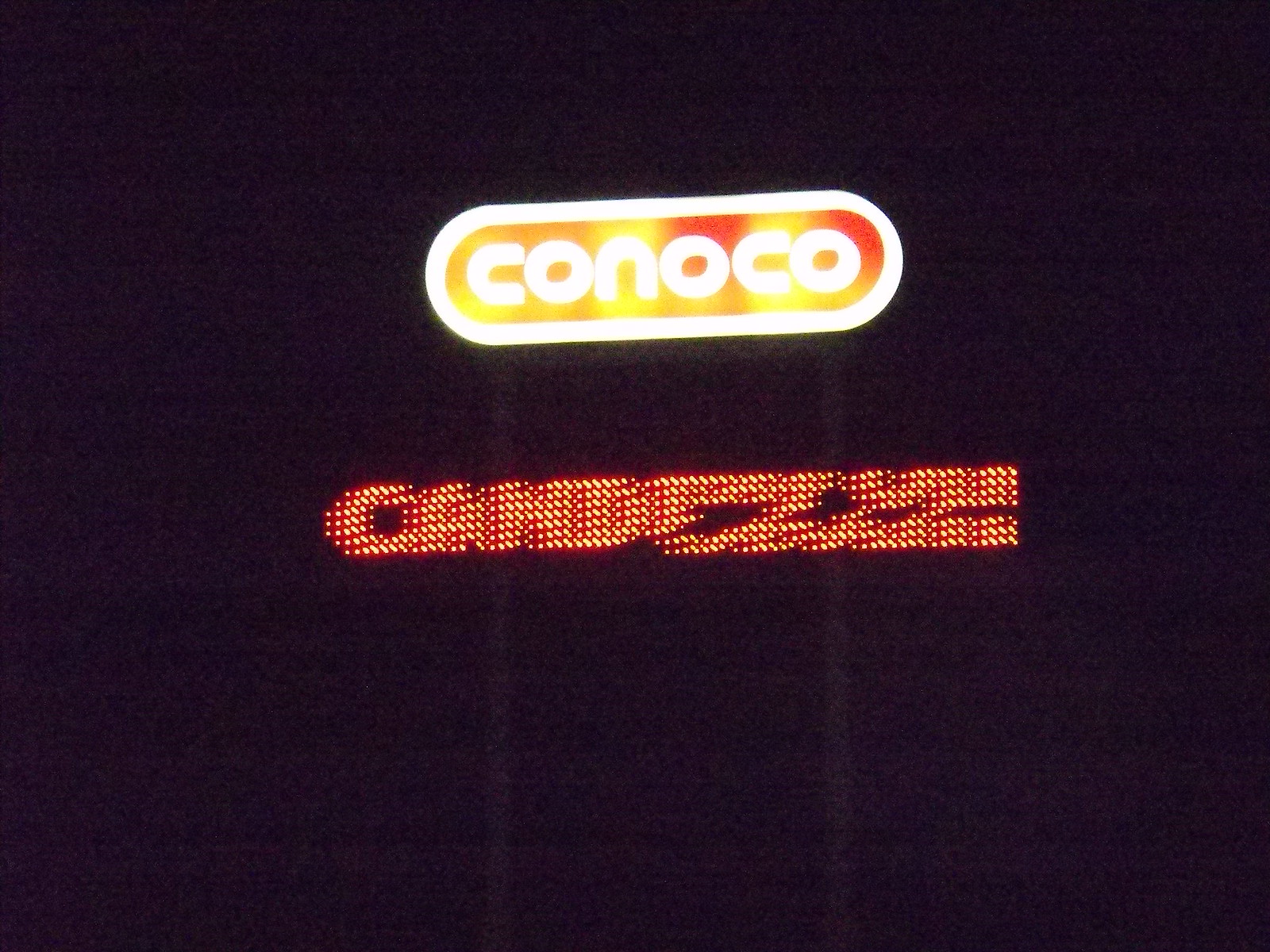Against the backdrop of a black night sky, this photograph captures two vividly illuminated signs mounted on parallel poles. The upper sign, an oblong shape bordered by white neon lights, prominently displays the word "CONOCO" in striking white neon letters set against a vertically striped red and yellow background. This vintage sign exudes a nostalgic charm, reflecting the classic design of mid-20th-century gas station signage. Below this, a smaller sign in red and yellow is also brightly lit. Though slightly less clear, it seems to spell out "Gradesa" in yellow neon lights, adding an additional layer of intrigue to the composition. The bright neon lights of both signs create a captivating contrast against the surrounding darkness, making them central focal points in the stark night scene.